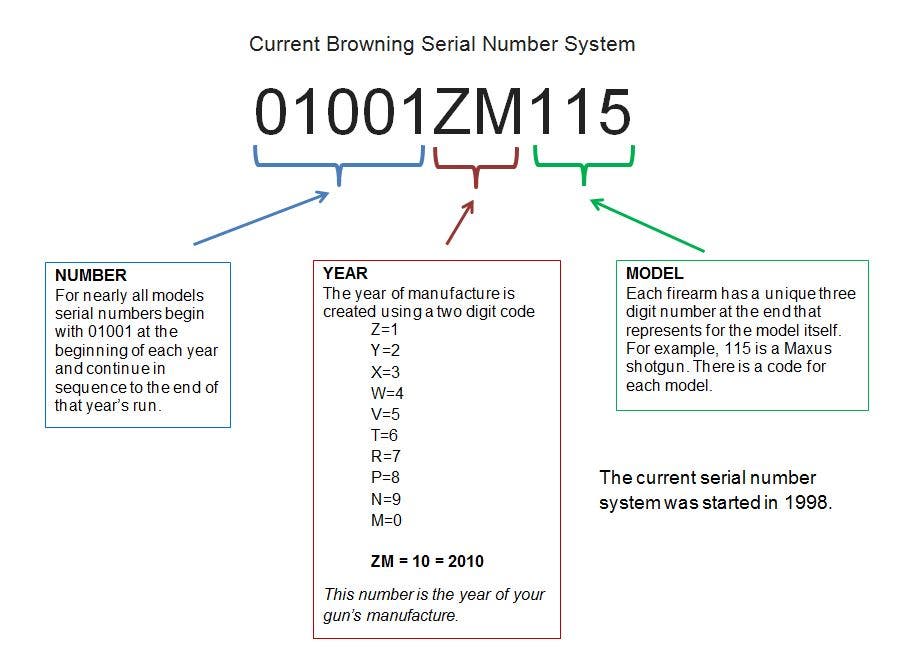This detailed landscape-oriented color infographic, set against a white background, illustrates the current Browning Serial Number System. Across the top, bold black text reads "Current Browning Serial Number System." Beneath, a prominent serial identifier "01001ZM115" is displayed. Below this are three color-coded brackets: blue, red, and green, each with arrows pointing to explanatory boxes.

The blue bracket, marked "Number," explains that serial numbers for nearly all Browning models commence with "01001" at the start of each year and sequentially advance until year-end. The red bracket, labeled "Year," clarifies that the manufacturing year is denoted by a two-digit code within the serial number, specifying the exact production year. Finally, the green bracket, titled "Model," states that each firearm’s model is represented by a unique three-digit number; for example, "115" corresponds to the Maxis shotgun. This system, initiated in 1998, ensures each serial number provides clear information on production sequences, year, and model type.